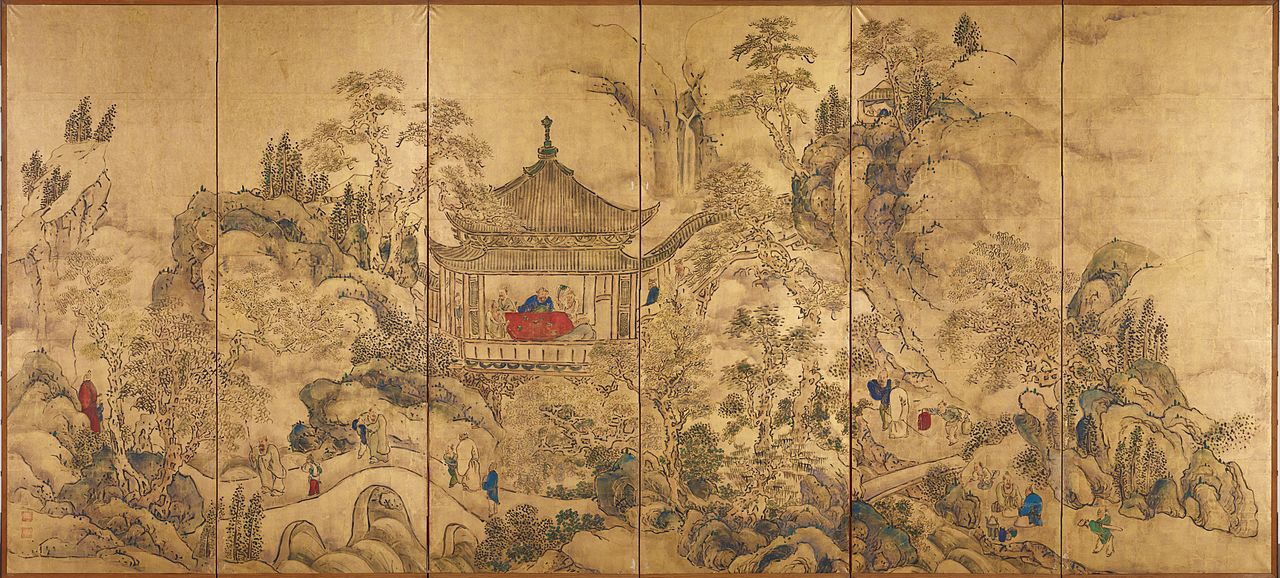The image showcases an ancient Chinese painting spanning six rectangular panels, predominantly executed in muted tones of black, white, brown, gold, and moss green. Central to the composition is an elaborate pagoda with a tall roof and open façades, resembling a stage adorned with a table draped in a red cloth. Among the figures within the pagoda, a person dressed in blue takes center stage, while another individual lies down nearby in red attire. The painting's landscape captures a serene scene with rocks, trees, and foothills, adding depth to the background.

In the foreground, scattered along a path, are several people clad in brightly colored robes, contrasting with the overall subdued color palette. Toward the left side, one individual wears red, while another on the far right is in green. The second panel features a figure with red clothing at the lower part, and the third panel highlights someone in blue. Additionally, the fifth panel presents both bright blue and red garments, enhancing the vibrant details of the scene. The final panel, showcasing a green-robed figure, completes the intricate and harmonious composition. The artwork remains unsigned, adding an air of mystery to its origin.